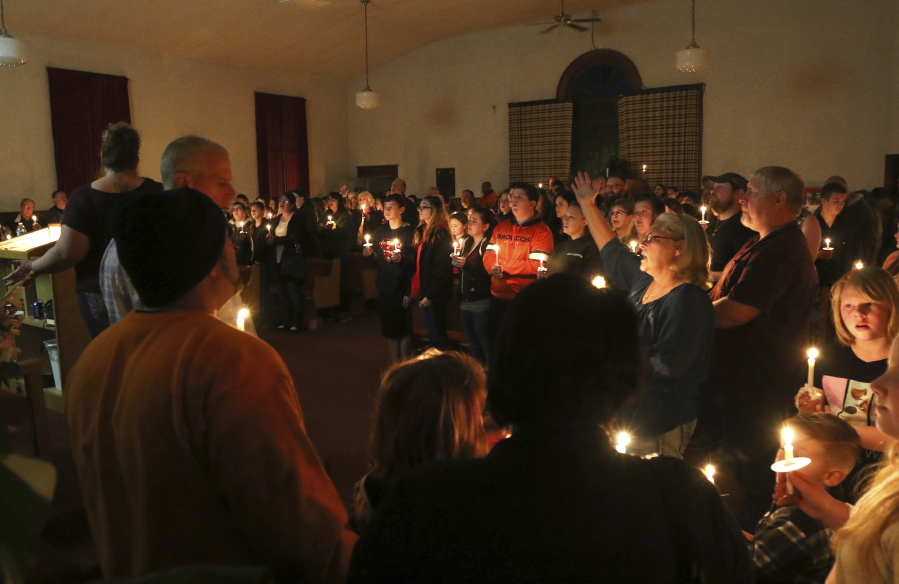The photograph captures a dimly lit indoor scene with a large group of predominantly Caucasian people, likely engaged in a communal or religious gathering, possibly a vigil or ceremony where they are holding lit candles. The room is spacious with a noticeable vaulted ceiling that forms a wide-angle V, painted in a soft yellow shade, a bit darker than the more tan-colored walls. 

On the left side of the image, the ceiling might arc slightly, and there are two dark-colored, vertically aligned rectangular wall hangings. Below these hangings, a pair of vertically aligned, mustard-yellow plaid curtains frame a black archway. The crowd is densely packed along the left wall and extends towards the center and right of the frame, becoming larger and more prominent in the foreground.

In the middle of the composition stands a central figure wearing a long-sleeved red shirt, surrounded by people in various colored clothing, including a woman in a blue long-sleeved shirt. Another notable figure in the foreground wears a black winter hat with a pom-pom, and beside them is a blonde woman or teenager. The silhouette of a man's short, curly hair is distinct on the far right. Another elderly male figure with spectacles and gray hair is visible behind the person with the beanie.

Lighting is minimal, primarily illuminated by the warm glow of candles each person is holding. There's a slight reflection of light on the left side, perhaps from a metal surface, and a podium is discernible to the left, suggesting a focal point or speaker's area. The floor, though faded in the dim light, appears to be light brown. The atmosphere suggests a solemn or celebratory occasion, where people may be singing, and some, including a woman with her arm raised, appear to be participating actively. The scene's overall ambiance is one of community and shared purpose within a humble, beige-painted room.